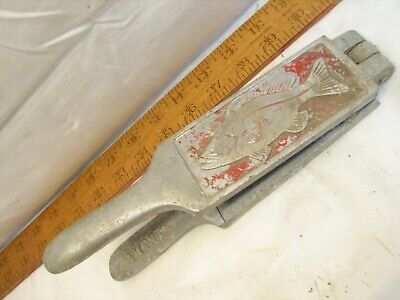The color photograph depicts a metal hinged tool, positioned centrally at a 45-degree angle, with its handles extending towards the top right. This tool, which appears to be a press or clamp, features two sections connected by a hinge. It is primarily silver, adorned with a raised image of a fish surrounded by partially peeled red paint. Adjacent to this tool is a section of a wooden yardstick marked with measurements from 23 to 30, though the units are unspecified. The yardstick, also angled at 45 degrees, overlaps behind the tool, and displays dark brown notches and lettering against its light brown surface. The objects rest on a white, plastic-covered background, with the bottom right corner showing part of the supporting surface. On the far left, a glimpse of what might be a wall is visible. The image captures the intricate details and colors of both the tool and the yardstick.